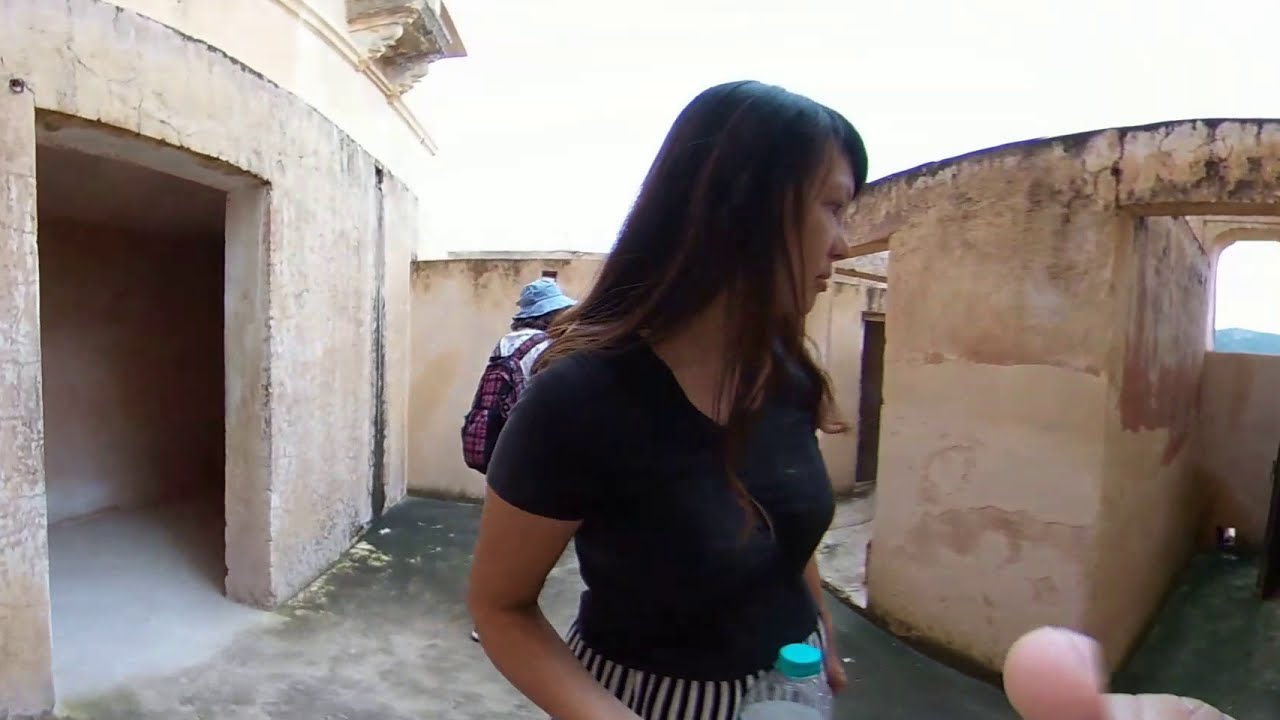The photo features a young Asian woman with long, dark brown, straight hair and bangs, standing front and center. She is wearing a black shirt and black and white striped shorts while holding a partially empty water bottle with a light blue top. She is looking to her right, seemingly observing an old stone structure with several rooms but no roof, suggesting ruins of a building that have likely been there for a long time. The ground is a mix of green, gray, and white, with some leaves scattered around. To the left, there's a large open door which is a beige and white color, while on the right, part of the building appears to be crumbling with an archway structure visible. Behind the woman, another person can be seen wearing a blue hat, white shirt, and red and black backpack, indicating a possibly touristic location with visitors exploring the ruins. In the distant background, a mountain and an overcast sky can be seen through a window.